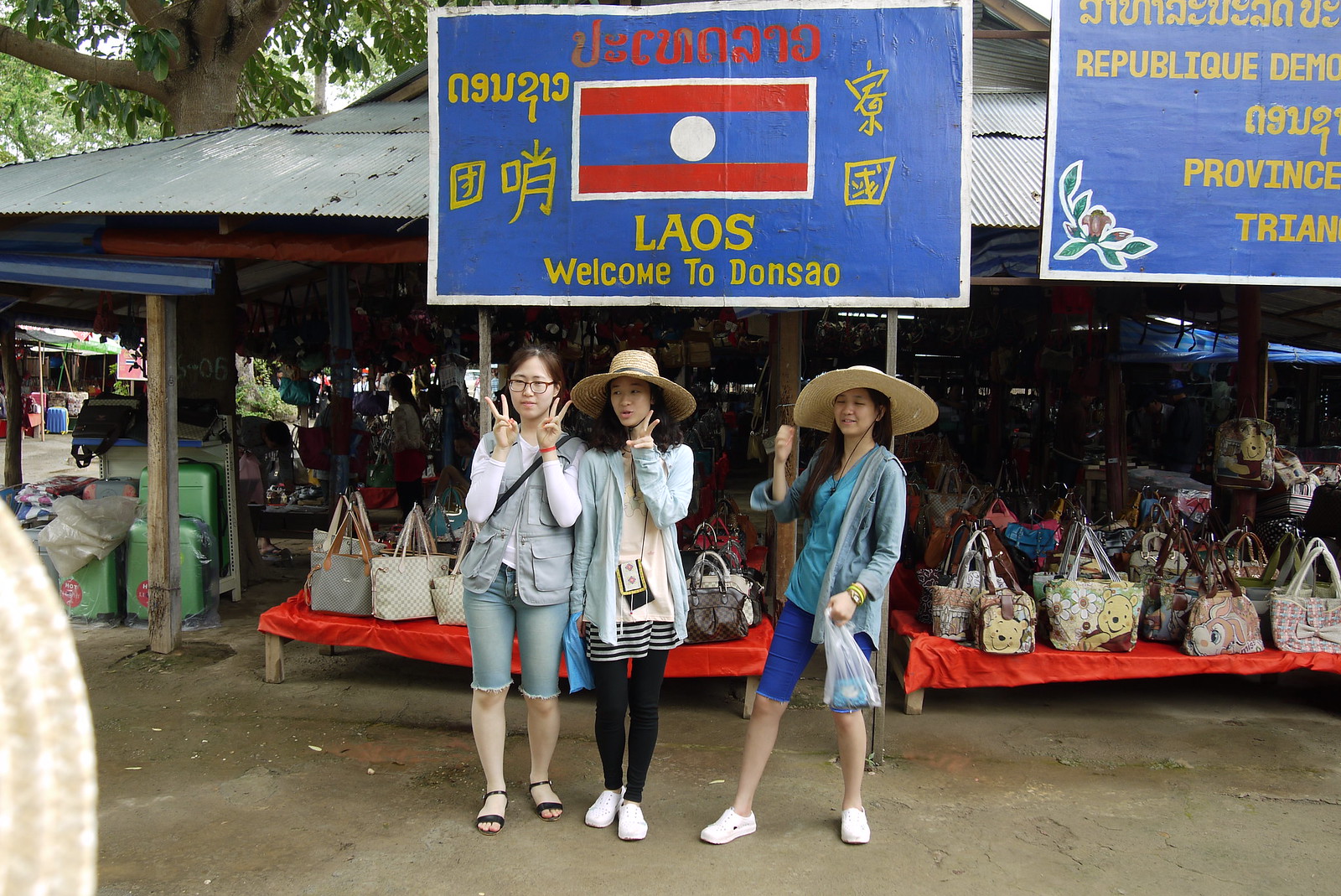This vibrant daytime photo features three female Asian tourists in Laos, posing energetically in front of a lively outdoor market stall that showcases a variety of accessories, including purses, wallets, and bags adorned with characters like Winnie the Pooh. They stand beneath a sign that reads, "Laos, welcome to Don Sao" in both Laotian and English, partially cut off with additional text that mentions "republic" and "province." The marketplace bustling in the background, filled with stalls under canopies, suggests a busy, colorful setting. The women, dressed in sun hats, shorts, and casual attire with colors like denim, black, cream, tan, pink, blue, and red, exhibit playful hand gestures—two flashing peace signs and the third caught in motion, slightly blurry. One woman sports glasses, and the group's dynamic poses add to the overall joyful and spontaneous atmosphere of the scene.